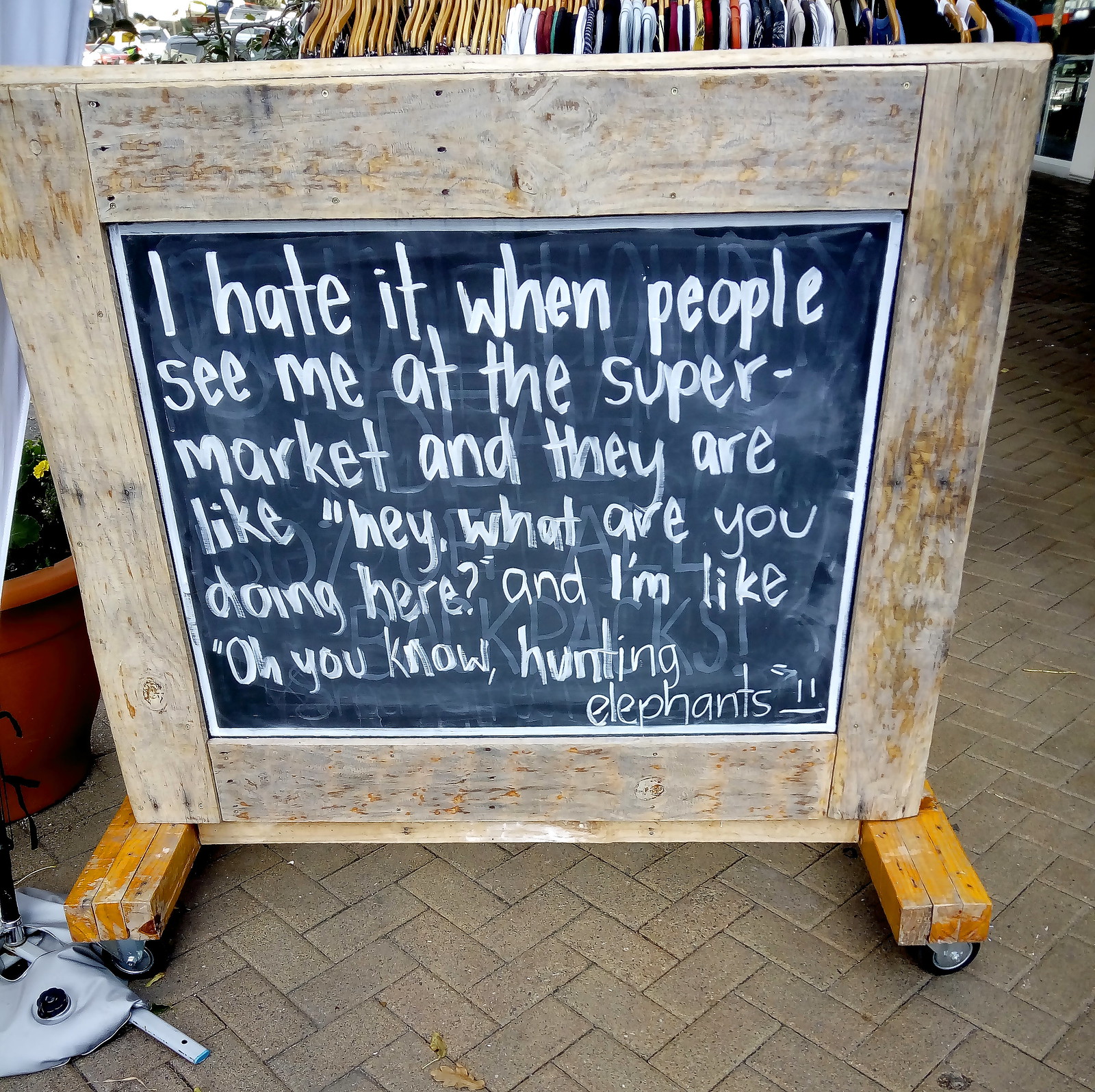The image depicts a rustic, square-framed chalkboard sign, mounted on a base with casters, situated on a brick courtyard floor. The chalkboard is surrounded by a wooden frame, showcasing a handwritten message in large, white chalk letters: "I hate it when people see me at the supermarket and they are like, hey, what are you doing here? And I'm like, oh, you know, hunting elephants." Below the text, a simple hand-drawn face with two eyes and a straight, unamused mouth is visible. The setting appears to be part of a market stall, with a rack of clothes hanging on hangers in the background and a plastic flower pot with a yellow flower positioned nearby. A parking lot with some cars is visible in the far left corner, enhancing the outdoor market atmosphere.